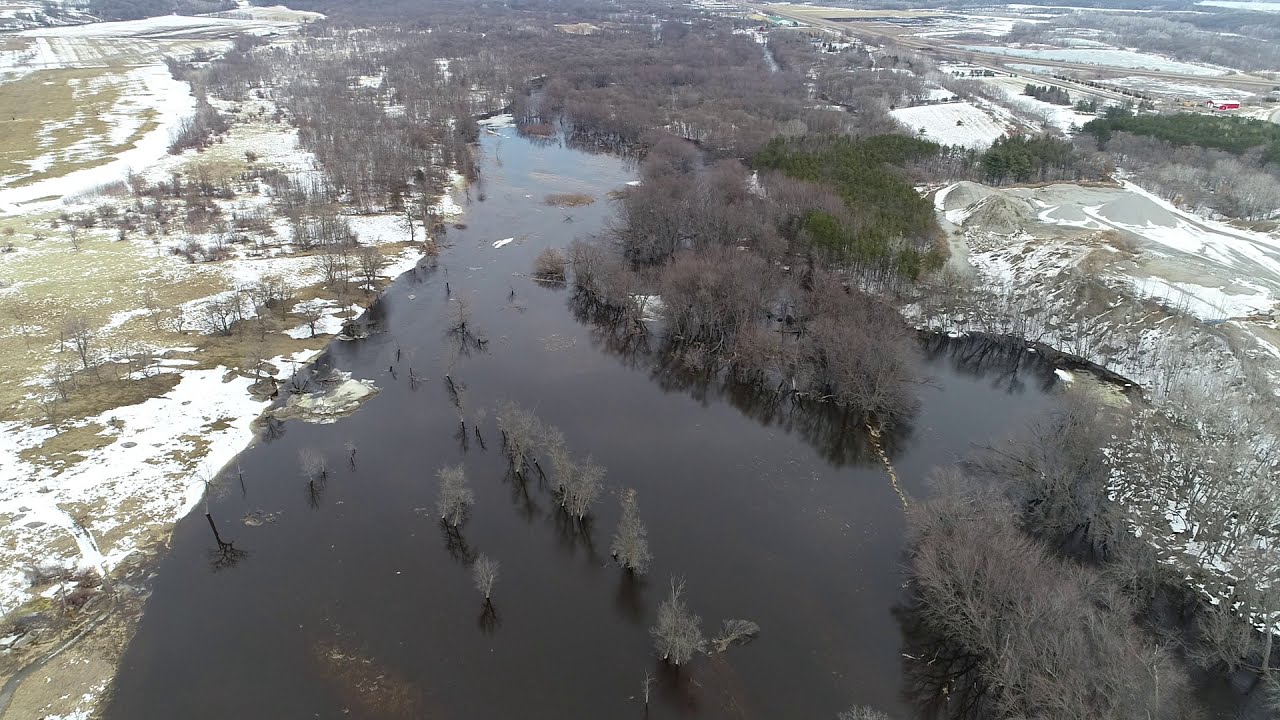The aerial image depicts a wintery, natural landscape dominated by a central body of dark, murky water, likely a river or stream, with trees growing intermittently from its shallow depths. The water, flowing upward in the image, is surrounded by snow-covered banks on both sides. To the left, patches of green grass covered by snow extend across fields scattered with trees and bushes. To the right, a mix of bare and green trees line the edge of the water, transitioning into a gravel or quarry area coated with snow around mounds of stone. Further out, the right side also features denser, light brown woodland and what appears to be a red building or farmhouse amidst the trees, with more green and grey fields stretching into the distance under daylight. The scene captures a rustic, tranquil environment with its natural elements and minimal human presence.